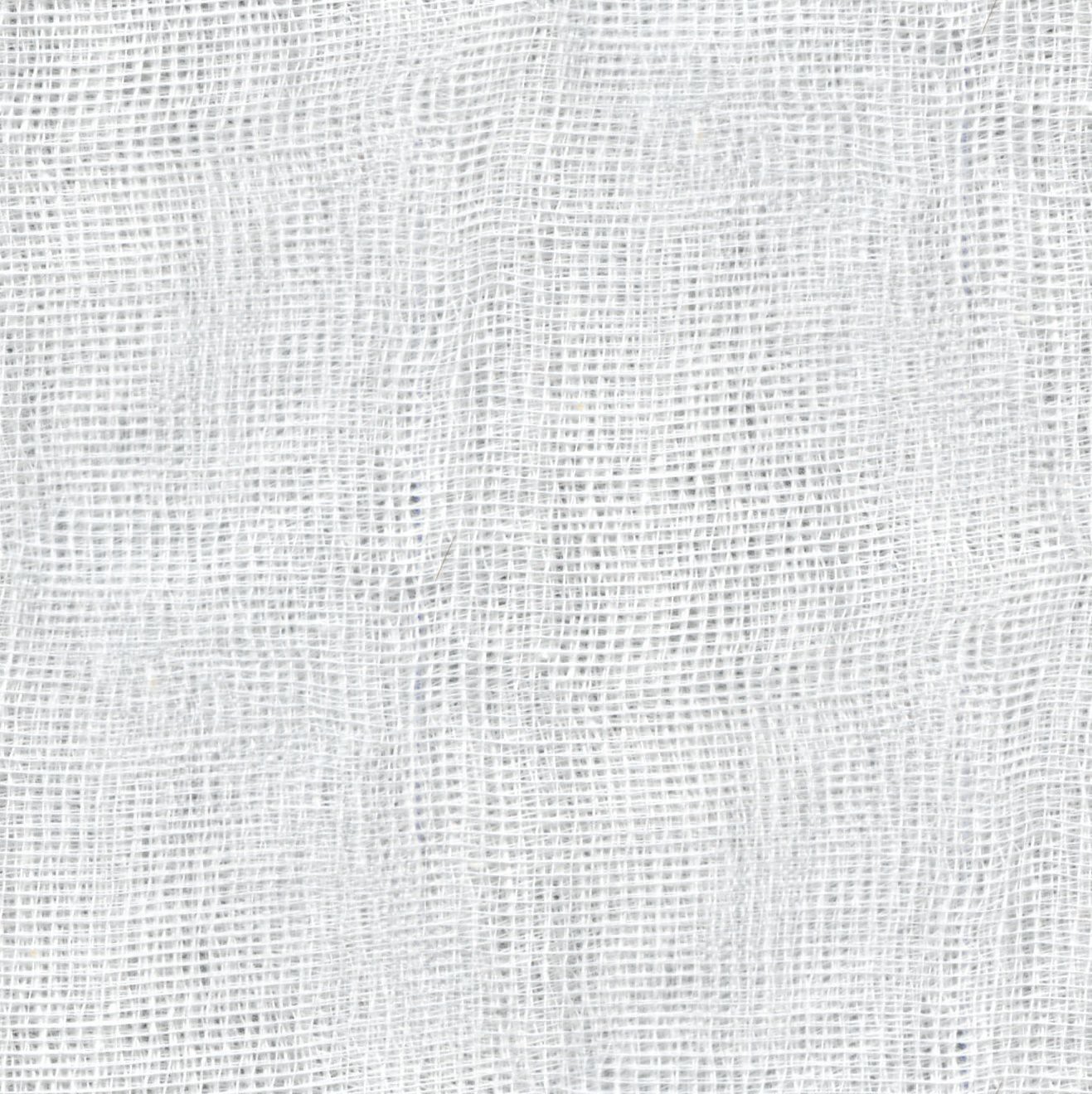The image depicts a close-up of what appears to be gauze fabric, filling the entire square frame of the photo. The gauze is composed of loosely woven, white cotton fibers arranged in a windowpane pattern. The soft material layers create subtle texture variations and crease marks, suggesting it has been folded. Lighting affects the photograph, introducing shades of gray and hints of blue, enhancing the intricate criss-cross weave of the threads. The gauze appears somewhat translucent, with small, airy squares that sometimes allow darker tones of gray or black to seep through, adding depth to the overall view.